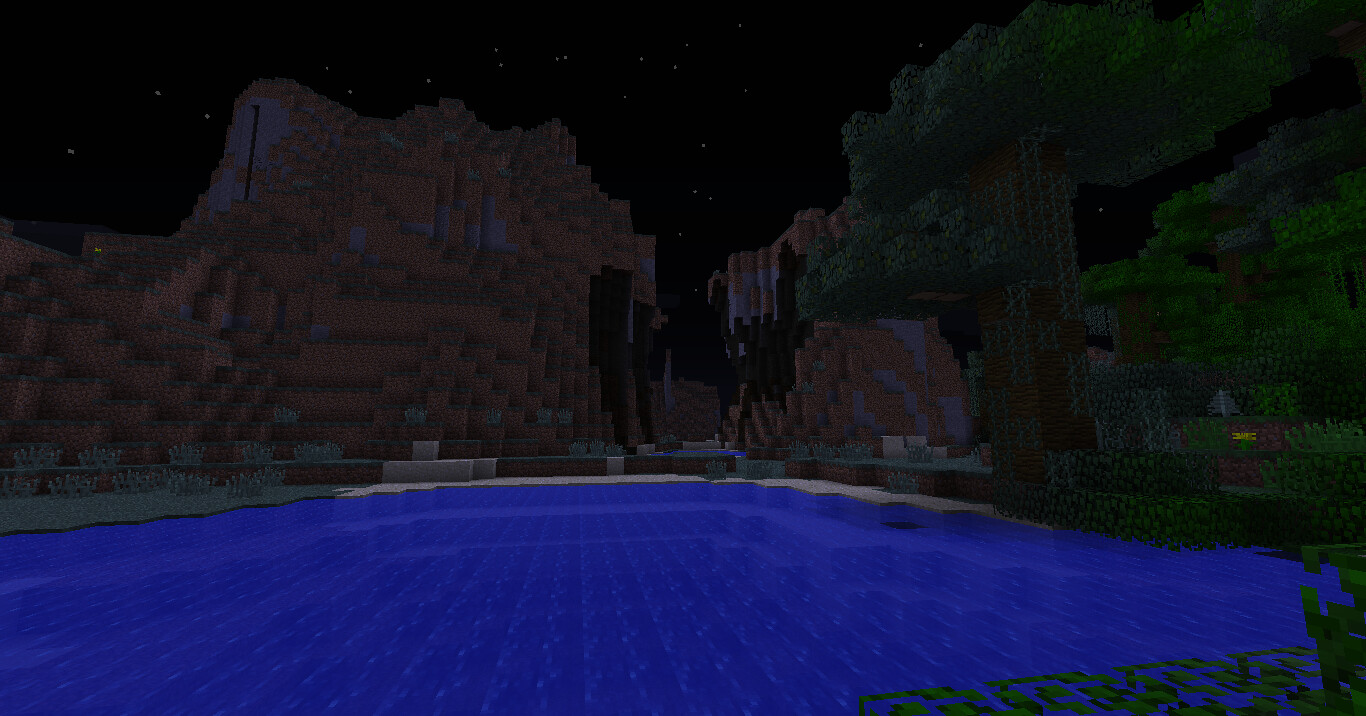This 3D-rendered image seems to capture a serene Minecraft nighttime scene. Dominating the lower third of the image is a large, deep, dark blue pool with stepped edges, hinting at a meticulously crafted swimming pool. Above the pool, the scene transitions into a brown and slightly purple cave-like structure, embodying the characteristic blocky texture of the Minecraft world. At the base of the cave, grey shrubs emerge, adding a touch of rugged flora. To the right, a cluster of trees and shrubbery stands tall, silhouetted against the dark sky. The night is clearly evident with a backdrop of deep black, sprinkled with small white dots representing distant stars. In the extreme foreground, the lower left corner reveals some greenery growing within the pool, adding a final touch of organic life to the tranquil scene.